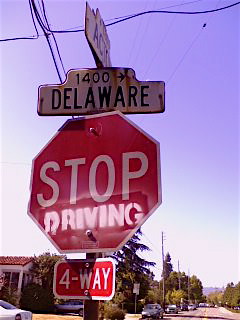This image captures an outdoor suburban scene centered around a prominently placed stop sign. The sky in the background transitions from a light purple at the top to a white near the horizon, setting a tranquil evening atmosphere. A mountain range or hillside is faintly visible in the distant background. The street is flanked by trees on both sides, and houses are visible to the left, with several cars parked along the road and in driveways.

At the forefront, a large red stop sign dominates the center of the image, with block letters spelling "STOP." Below, the word "DRIVING" is spray-painted in a different font, making the sign read "STOP DRIVING." Beneath this, a smaller rectangular plaque indicates it's a four-way stop with the words "4-WAY." Above the stop sign, a street sign reads "1400 Delaware," while a second, obscured sign starts with "A-C" but is unreadable due to its angle. Overhead, electric wires crisscross the sky, further framing the scene. To the left of the stop sign stands a pine tree, adding to the suburban feel. The road descends slightly to the right, lined with more parked cars extending into the horizon.